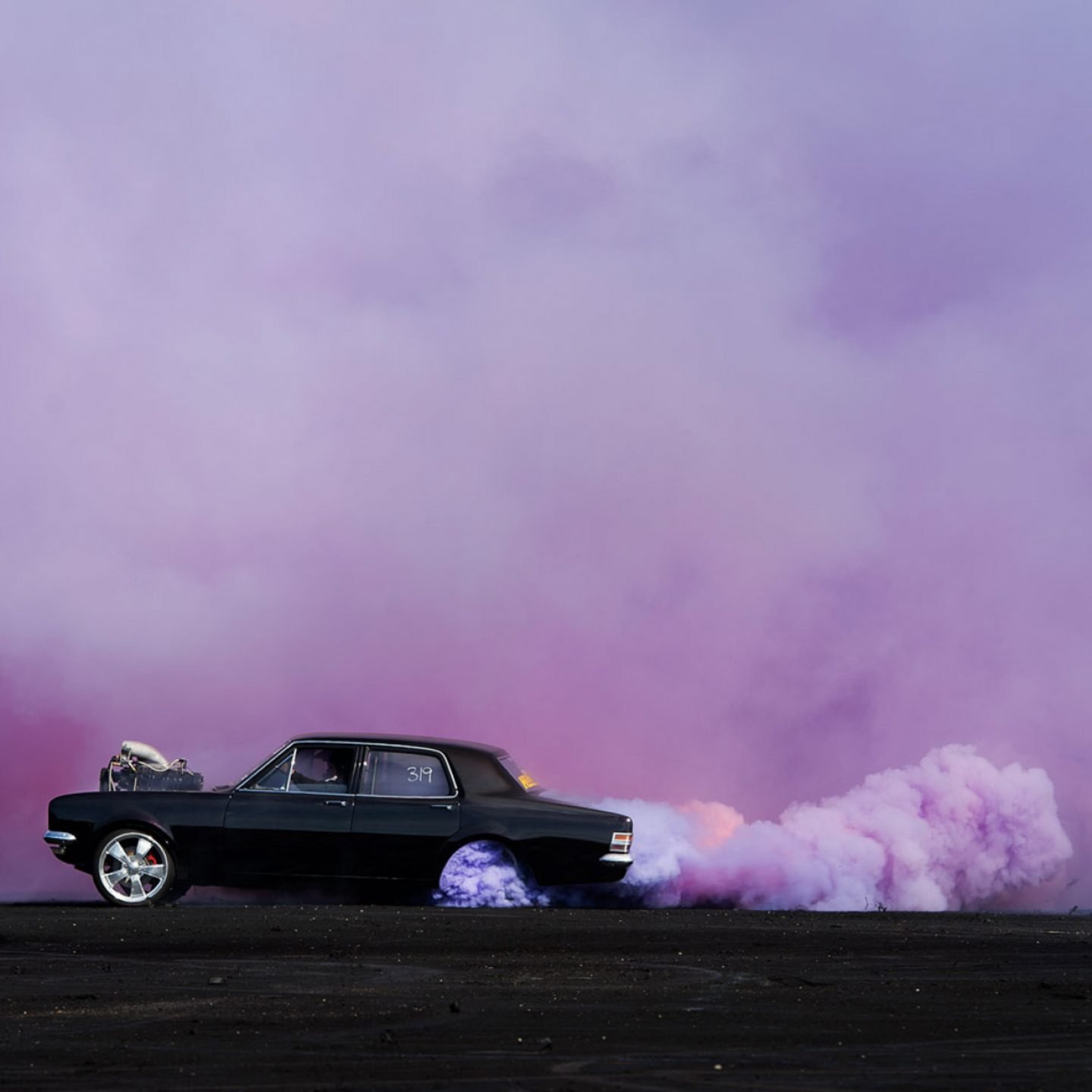The image is a large digital photograph, slightly taller than wide, showcasing a dramatic scene set against a sky filled with clouds of white and purple. The focal point is an older style black four-door sedan prominently occupying the lower left portion of the frame. The car's left side faces the viewer, with the number "319" clearly visible in white on the back window. The vehicle's engine appears to be protruding from the raised hood, adding a sense of raw mechanical power. Purple-tinged smoke billows dramatically from both the rear left wheel and the back of the car, creating a striking contrast with the black asphalt beneath. The driver, barely visible, adds a touch of intrigue by wearing a cowboy hat.